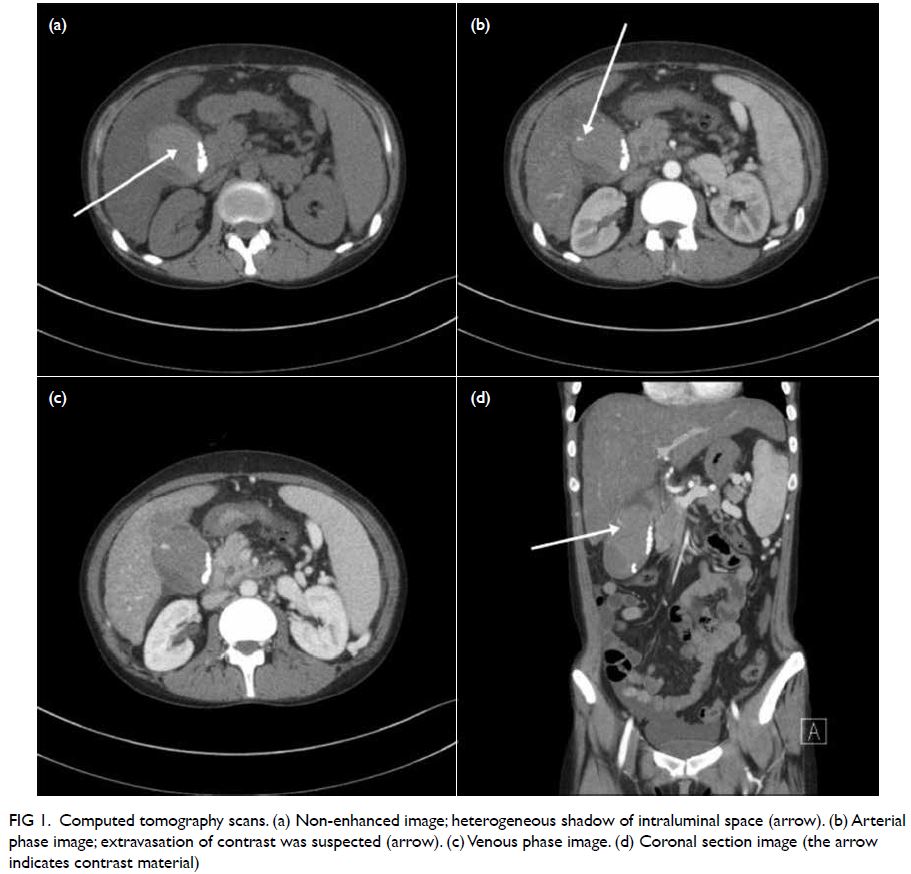This image displays four detailed computed tomography (CT) scans, labeled A, B, C, and D, each highlighting different phases and features. The scans are arranged in quadrants against a black background, with each image having its unique focal points and annotations indicated by arrows. 

- **Image A (Top Left)**: A non-enhanced scan showing a heterogeneous shadow within the intraluminal space, marked by an arrow, likely exhibiting brain features given the oval shape and lobe areas.
- **Image B (Top Right)**: An arterial phase image with an arrow pointing to a section where extravasation of contrast is suspected, suggesting an area of particular diagnostic interest.
- **Image C (Bottom Left)**: A venous phase image, providing further detail as part of the scan series.
- **Image D (Bottom Right)**: A coronal section image, distinguished by an arrow indicating contrast material, and potentially showing the torso of a person.

At the bottom of the display, text on a white background clarifies the images as "Figure 1: Computed Tomography Scans," with additional annotations describing each scan phase and highlighting specific diagnostic features.